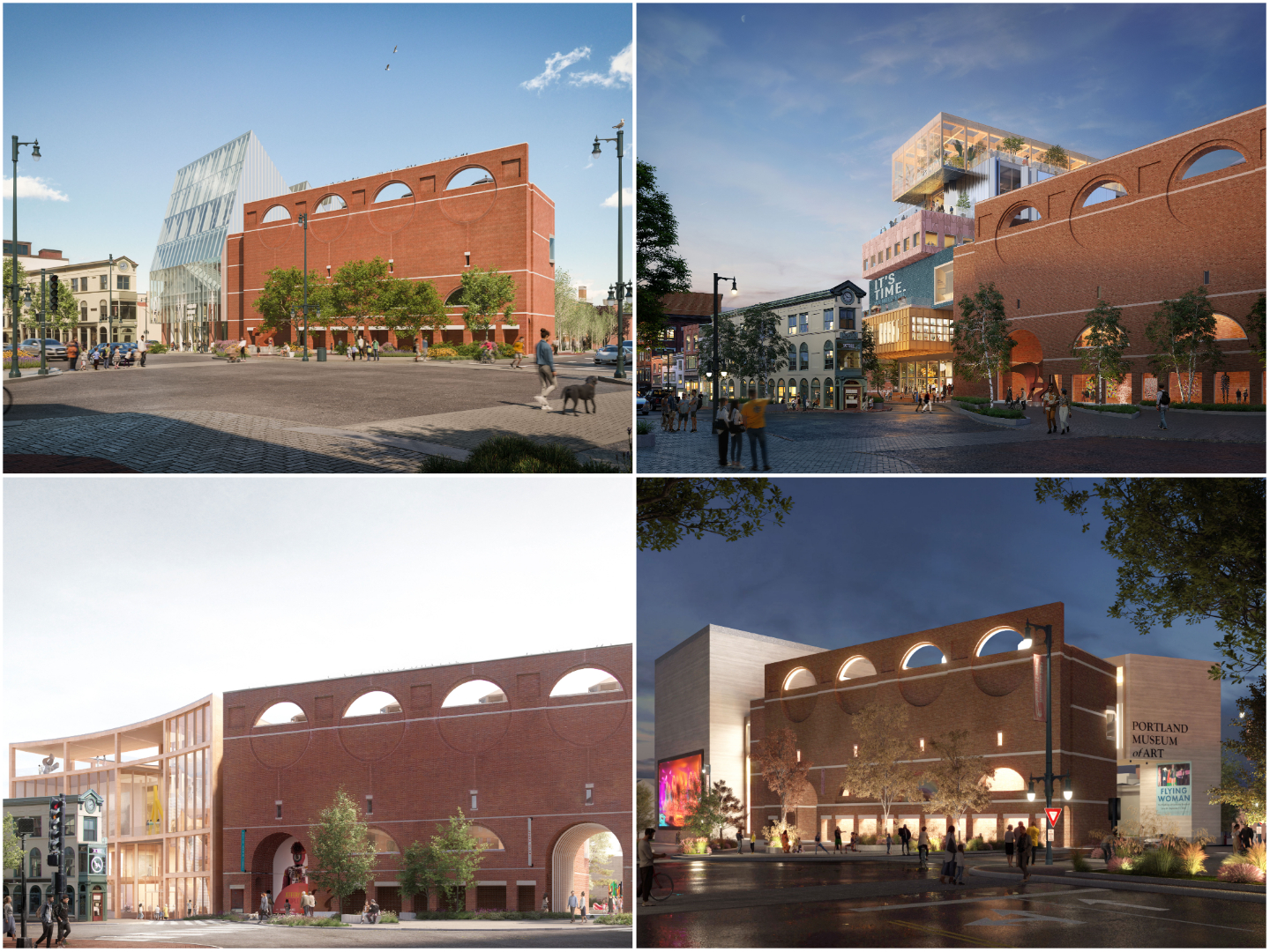The image is a collage featuring four exterior shots of the Portland Museum of Art, each taken at different times of day. The top left photo displays the museum during an early morning or possibly a cloudy day, revealing a tall white building with an odd shape next to the main brick museum building, which is characterized by four open semicircles at its top and surrounded by some trees. The upper right image might be during sunset, capturing a different side of the building that includes a narrow structure with a clock atop it. The bottom left photo presents another daytime view, centering more clearly on the brick facade and its distinctive half-moon shapes, with a neighboring glass building and cobblestone street. Lastly, the bottom right shot is taken at night, highlighting the external lighting that accentuates the building's architectural details, including neon signage in the left corner that emits red, orange, and blue hues. In all shots, blurred figures of people and pets can be seen in the background, adding life to the scene while emphasizing the museum's imposing presence and design.